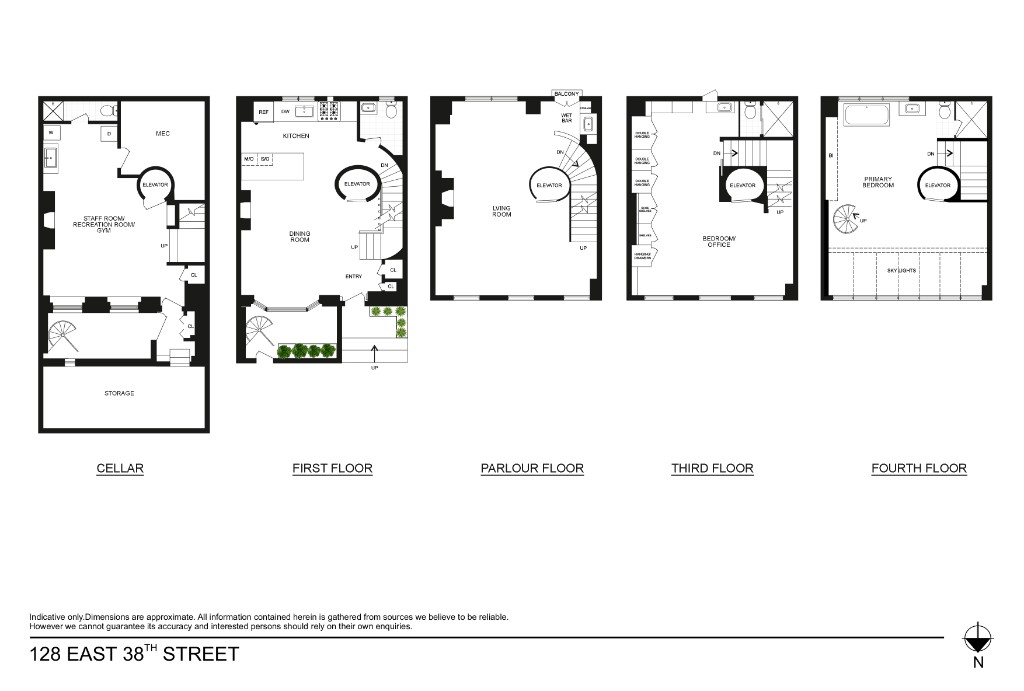A detailed architectural floor plan set on a white background showcasing five distinct floors of a house located at 128 East 38th Street. The layout, arranged from left to right, includes a spacious cellar floor, the first floor, the parlor floor at the center, the third floor, and the fourth floor. Each floor is meticulously labeled, offering insights such as a bedroom office, separate bathrooms, a living room, and a dining room positioned on different levels. Predominantly in black and white, the plans also feature touches of green to indicate landscaping. Beneath the plans, small, illegible text is followed by a clarifying line, with the address prominently displayed. An arrow pointing down, accompanied by the letter 'N', is situated at the right end of the bottom section, suggesting orientation.